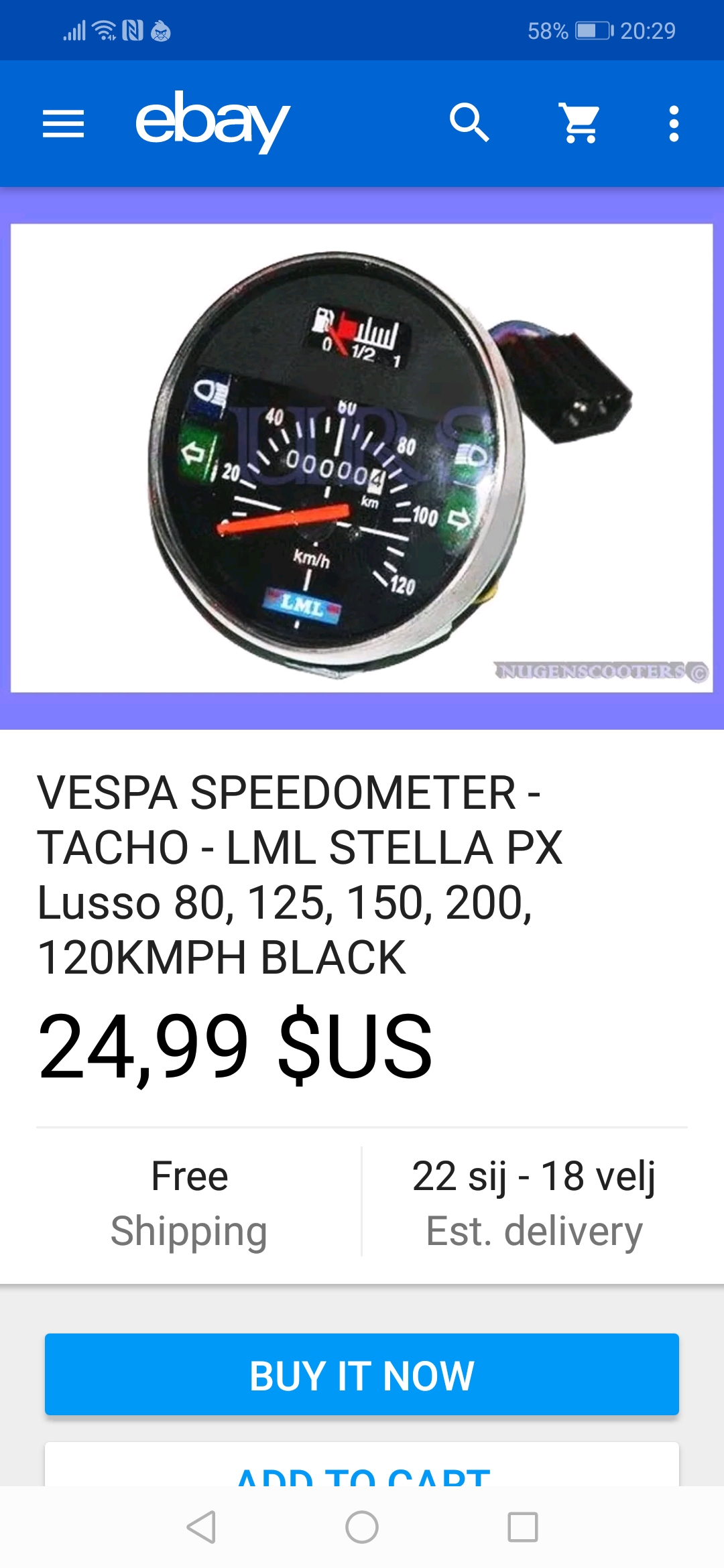In this photograph, we see a screenshot of an eBay auction listing captured from a cell phone. The phone's status bar at the top indicates a battery life of 58% and the time is 20:29. The eBay mobile interface is visible with icons for search (a magnifying glass), cart (a shopping cart), and additional options (three vertical dots) positioned at the top right.

The central feature of the listing is a speedometer, which appears versatile enough for use with a bicycle, motorcycle, or car. The speedometer has a black base and includes a gauge for measuring speed in kilometers per hour. The product description reads: "Vespa Speedometer, Taco, LML, Stella PX, Lusso, 80, 125, 150, 200, 120 kilometers per hour black". The listed price is $24.99 USD, and the item comes with free shipping.

To the right, there is a notation "22SIJ-18VELJ" and an estimated delivery date. At the bottom of the listing are options for immediate purchase with a blue "Buy It Now" button, or adding the item to the cart with a white "Add to Cart" button. 

Additionally, navigation buttons at the bottom of the screen allow users to move back, go home, or close the app. This detailed screenshot vividly depicts the user interface of eBay on a mobile device, showcasing the specific product and purchasing options available.